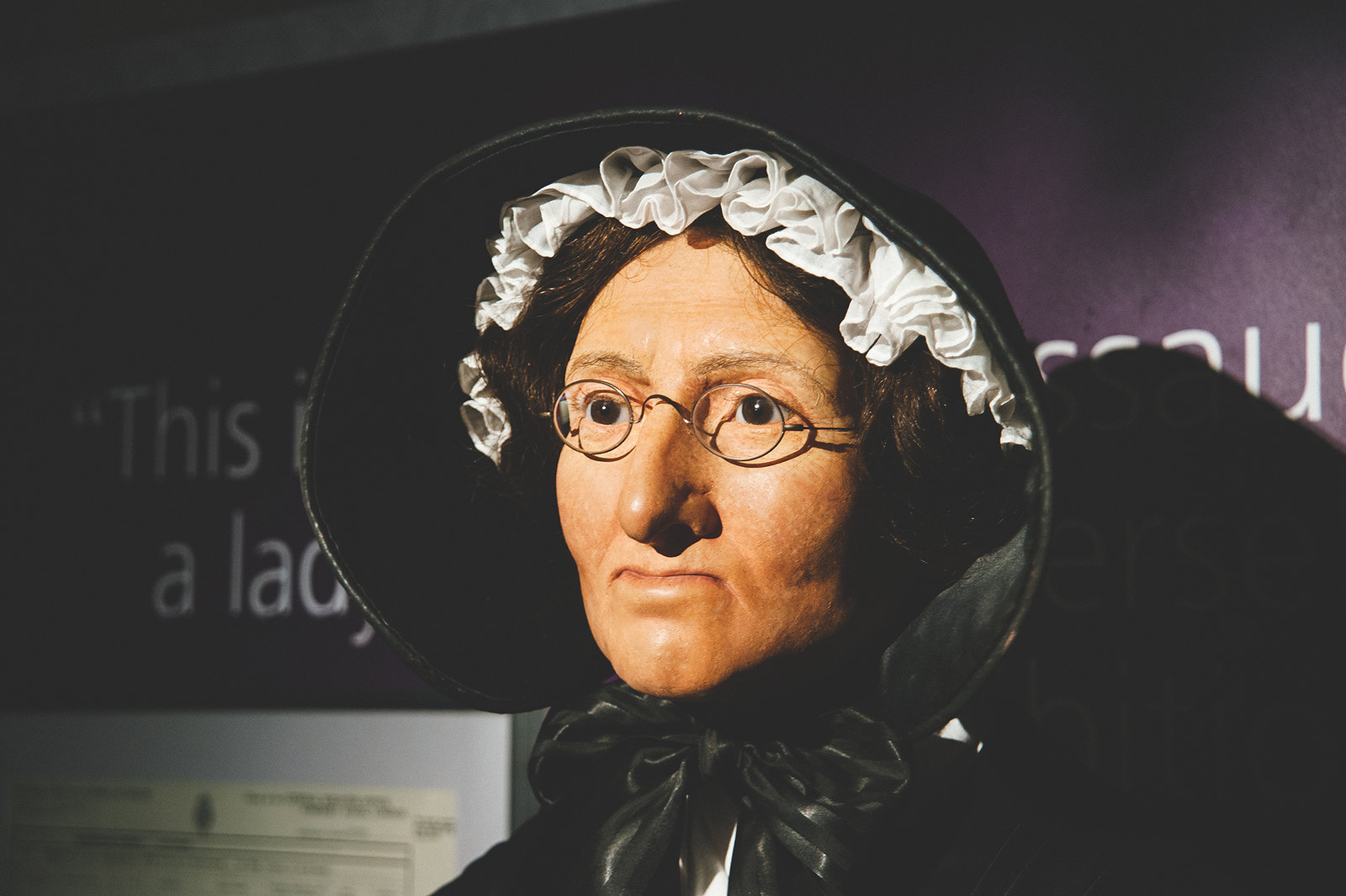The image depicts an eerily realistic figure of an elderly woman, who could be mistaken for a meticulously crafted wax mannequin. She wears small, wire-rimmed glasses perched on her nose, framing her stern, dark brown eyes which gaze intently from right to left with an unhappy expression. Her face is framed by short, brown hair hidden beneath a black bonnet adorned with white, ruffled cotton. A black ribbon is tied around her neck, complementing her black top, which obscures much of her body. The background is a dark gray or purple wall with white text partially obscured by her head, appearing to read "this is a lady." Additionally, there is a white rectangular piece of paper with printed text that is blurry, situated in the lower left-hand corner. The scene is illuminated by a bright light, casting a shadow behind her and accentuating her stern, pilgrim-like appearance.